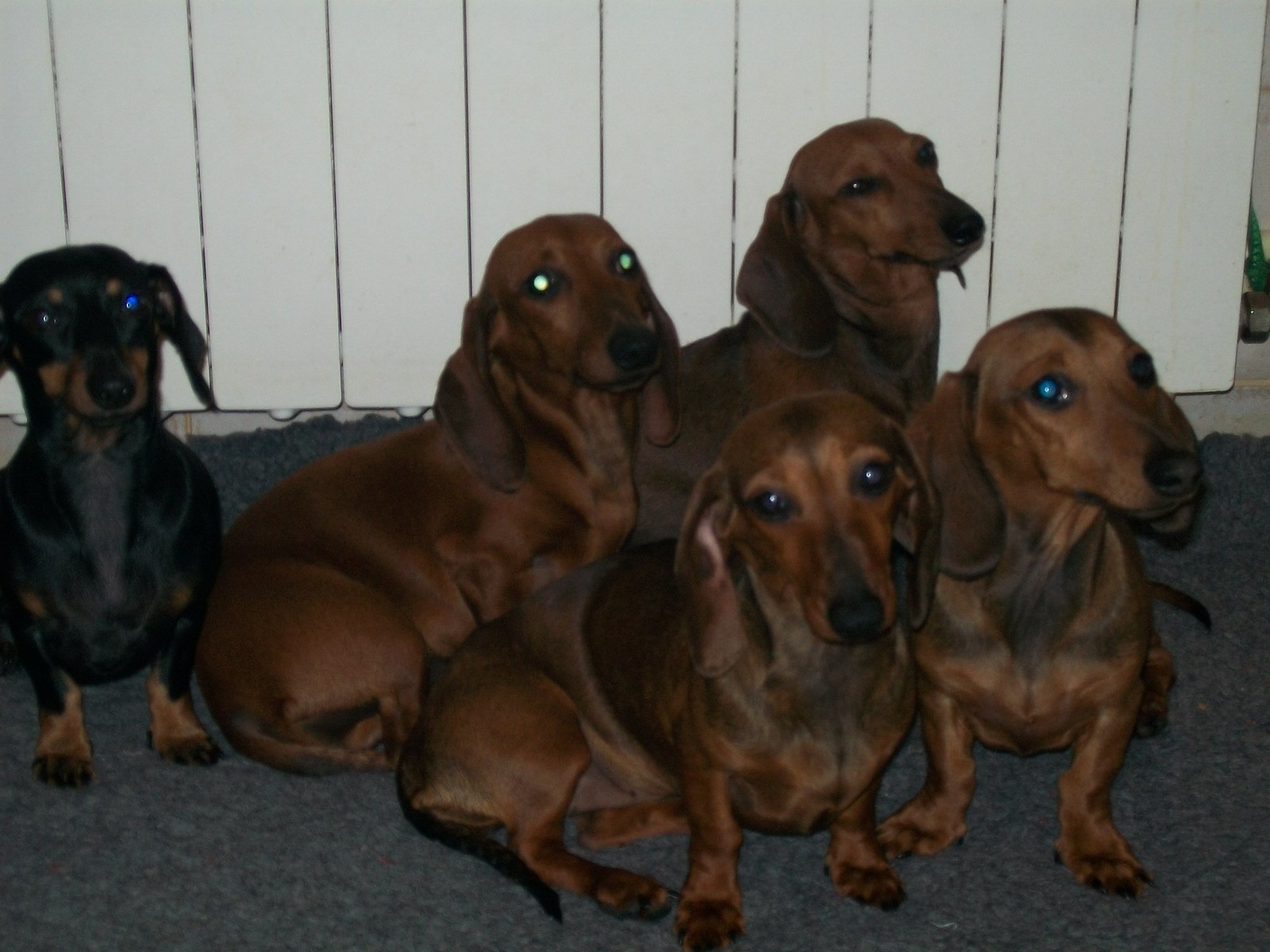In this image, there are five small dachshunds resting on a dark gray carpet in front of a wooden wall made of vertical slats. The dachshunds are mostly chocolate brown in color, with the exception of one black dachshund with distinctive brown markings on its paws, muzzle, and above its eyes. The black dachshund sits to the left, facing the camera. The other four dachshunds, also turned towards the camera, display various shades of chocolate brown. They are arranged in two rows: the dachshund closest to the black one is lying sideways with its chest to the right and head facing the camera, another is lying down with its chest to the right behind the first, one is sitting behind the previous dog with its head slightly raised, and the last one is positioned on the far right, facing directly towards the camera with a slightly turned head. The wooden wall behind them adds a rustic backdrop to the scene, suggesting a cozy indoor setting for these clearly cherished pets, likely belonging to a dachshund enthusiast.